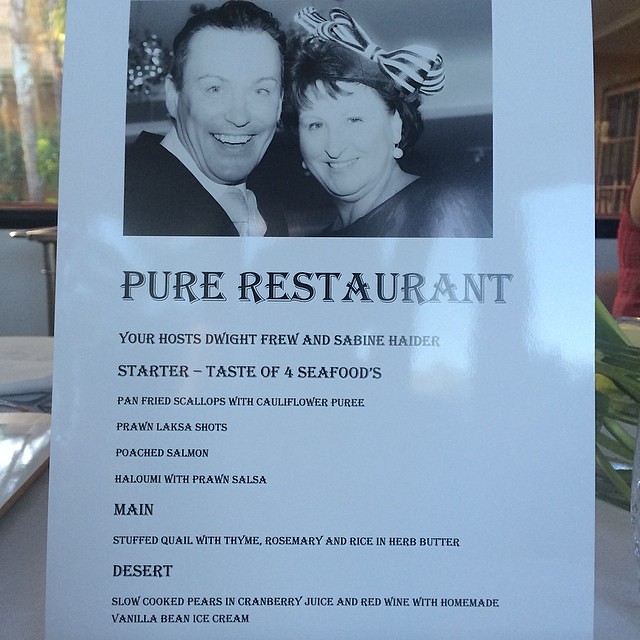The image showcases a menu for an event, likely a wedding, held at Pure Restaurant. The menu is elegantly placed on a table, complete with plates and utensils in the background. At the top of the menu, there is a black and white photograph of a smiling couple, possibly the hosts or celebrated guests, dressed in what appears to be vintage 1950s or 60s attire—the man in a suit and the woman in a black dress with a hat featuring a large bow. The menu details an exquisite dining experience provided by hosts, Dwight Frew and Sabine Hayden, featuring starters like pan-fried scallops with cauliflower puree, prawn laska shots, poached salmon, and halloumi with prawn salsa. The main course highlights stuffed quail with thyme, rosemary, herb butter, and rice. Desserts include slow-cooked pears in cranberry juice and red wine paired with homemade vanilla bean ice cream. The setting behind the menu suggests an inviting interior space with a bookshelf, a peach-colored tank top visible on a person to the right, and a glimpse of a window with a tree outside, adding a cozy and intimate ambiance to the scene.